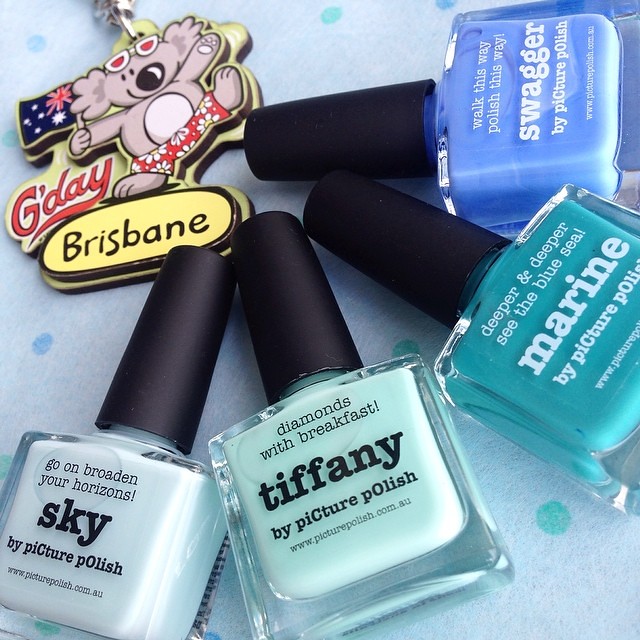The image showcases a collection of beauty products framed predominantly by a set of four Picture Polish nail polishes, each distinct in name and color, arrayed in a semicircle. At the top left, there's a whimsical keychain from Brisbane featuring a cartoon koala in red and white floral board shorts, sporting red and white sunglasses. The koala is joyfully holding an Australian flag and beneath its left arm, text reads "G'Day Brisbane!”

Starting from the bottom left, the first nail polish bottle is labeled Sky, a delicate pale blue shade with the tagline "Go On, Broaden Your Horizons". The next bottle, positioned above and to the right, is Tiffany, a soft greenish-blue evoking Tiffany blue, with the phrase "Diamonds With Breakfast". Moving further right is Marine, a deeper greenish-blue shade accompanied by the description “Deeper and Deeper, See the Blue Sea”. The final bottle, located at the top right, is Swagger, a vibrant purplish-blue marked with “Walk This Way, Polish This Way”. All nail polishes have a consistent design - glass bottles with black screw-on lids, and are part of the Picture Polish brand, available at PicturePolish.com.au.